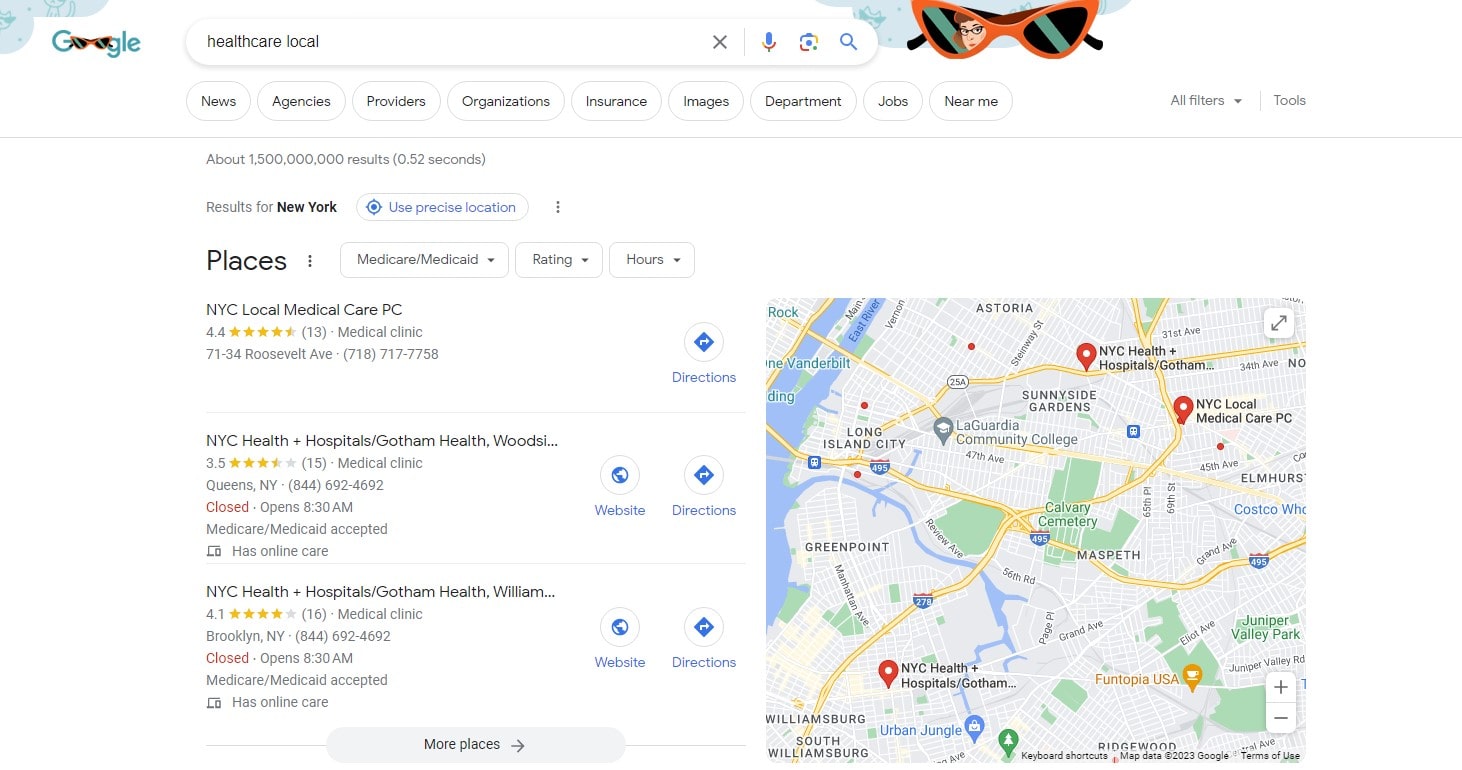In the image, the top left corner prominently features the word "Google," displayed in a greenish-blue color, with the letters G, the second G, and LE all in this shade. Notably, the double O's are creatively replaced with the shape of sunglasses. To the right of this logo, within the search bar, the text "Healthcare Local" is visible. On the right side of the search bar, there are several icons: an X symbol, a microphone symbol, a photo symbol, and, at the very end, a magnifying glass icon.

Beneath the search bar, there are several categories listed horizontally from left to right: the first category, slightly blurred, appears to be "News," followed by "Agencies," "Providers," "Organizations," "Insurance," "Images," "Department," "Jobs," "Near Me," and on the far right, "AI Filters and Tools."

Centrally located in the image is the word "Places," next to which are three boxes labeled "Medicare," "Rating," and "Hours." Below this section are three links: "NYC Local Medical Care," "NYC Health," and "NYC Health + Hospitals."